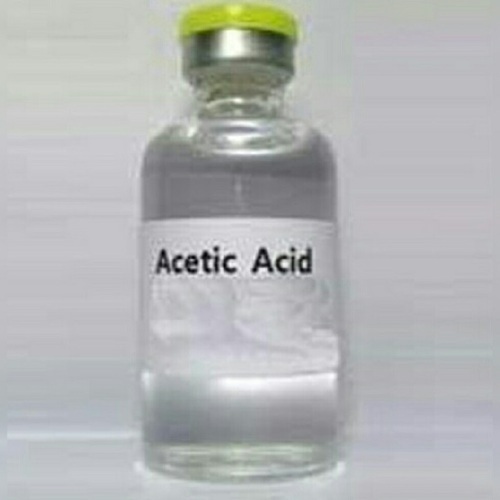The image depicts a small, clear glass vial of acetic acid, filled almost to the top with a clear liquid that resembles water. The vial features a white label with black, sans-serif text that reads "Acetic Acid," with both 'A's capitalized. Under the text, the label has a cloudy or swirled gray design. The top of the vial is wrapped with a silver band, leading up to a lime-green lid that adds a bright, contrasting element. The vial is placed on a white surface, which blends seamlessly into the white background, highlighting the transparency and clarity of both the vial and its contents.